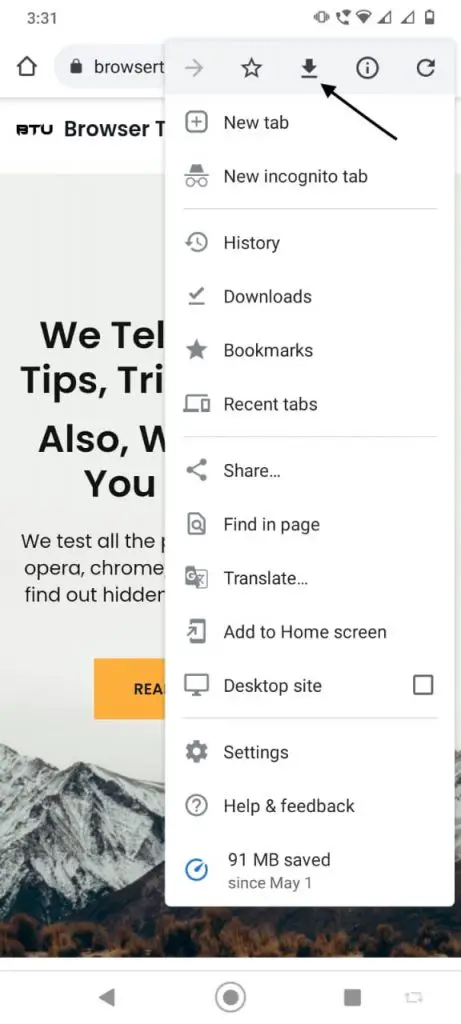The image is a screenshot with a white background. At the top-left corner, the time is displayed as "3:31" in gray. The battery, Wi-Fi, and reception icons are located in the upper right-hand corner. On the left side, two rows down, there is a house icon outlined in black, next to a long gray oval. Within this oval, there is a filled-in black lock icon on the left, followed by the word "browser." 

A box has opened up over the text following the word "browser," displaying a long rectangle with various icons and text. The top row of icons in this box includes a right-pointing arrow, a star, a download symbol, an eye inside a circle, and a reload icon. Below these icons, there is a list of options: "new tab," "new incognito tab," "history," "downloads," "bookmarks," "recent tabs," "share," "find in page," "translate," "add to home screen," "desktop site," "settings," "help and feedback," and "91MB saved."

To the left of this box, there is a section with a light gray background, partially showing text that includes "we," "T-E-L," "tips, T-R-I," "also, W," and "you." This text appears cut off at various points. At the very bottom left of the image, there is a partially visible snow-covered mountain. The lower part of the image from the middle to the right and along the bottom edge is filled with a brown color.